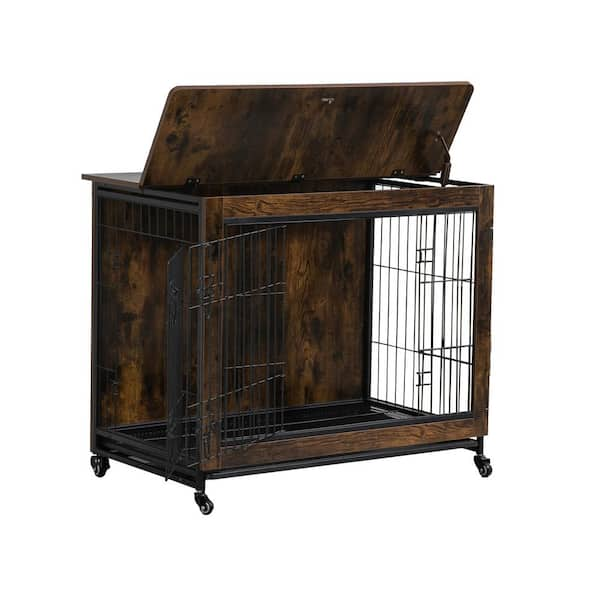In this detailed color photograph, taken in landscape orientation against a solid white background, the subject is a portable rectangular cage that resembles a piece of furniture, perhaps a dog crate. Constructed from dark wood and featuring a black iron grid work, the cage has a sophisticated and sturdy appearance. The front of the cage showcases two doors with latches, one of which is fully opened to the left while the other remains partially closed and secured by top and bottom latches. The side sections feature similar open-grid designs, offering good ventilation. The hinged lid on the top has been opened at an angle, pointing diagonally to the top right of the image. Inside, a black plastic tray lines the bottom to catch any mess. The entire unit stands on four caster wheels, making it easily movable. The back of the cage is a solid dark brown wood panel. This image, in the style of photographic representational realism, emphasizes the practical and aesthetic features of this versatile cage.